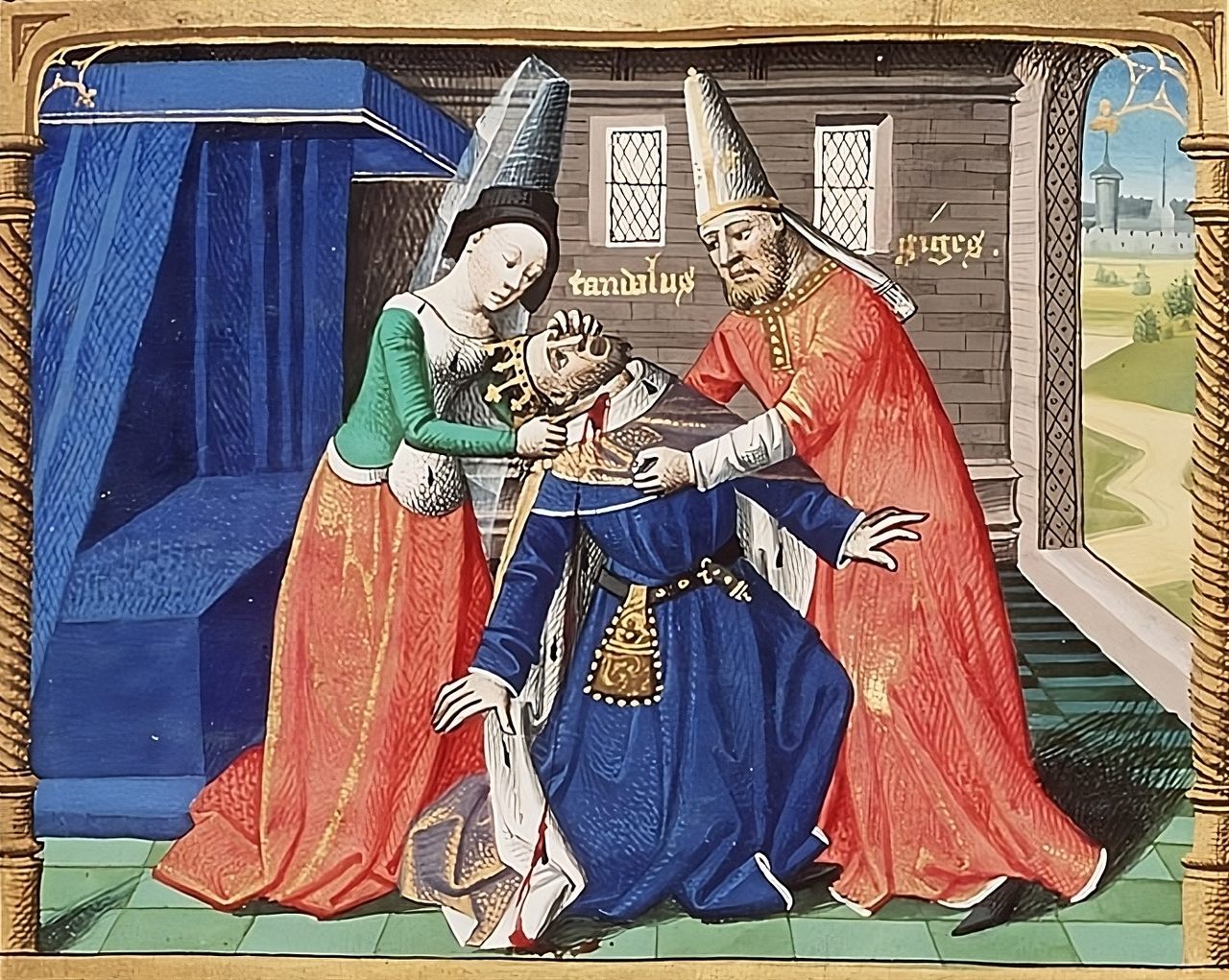This is a detailed medieval-style painting framed with a gold-like border mimicking wood. It depicts a dramatic scene taking place in a medieval room adorned with brown walls and a blue-canopied bench to the left. 

At the center of the image, three figures stand out. On the left, a woman dressed in a green long-sleeved blouse and an orange skirt that reaches the floor, accentuated by a tall black conical hat, is actively engaged in the scene. Beside her, to the right, stands a man wearing an orange robe and a cream-colored pointed hat, also participating in the unfolding drama. Between them, a figure dressed in regal attire—a blue robe and a gold crown—identifies him as a king. 

The woman's hand grips a small, sharp knife pressed to the king’s neck, from which blood visibly trickles down, staining his white collar. The king appears to be fainting or succumbing to his injuries, his head tilting back towards the woman. This intense and emotive scene captures a moment of betrayal and violence, all within the confined, period-accurate room, providing a stark atmosphere to the narrative.